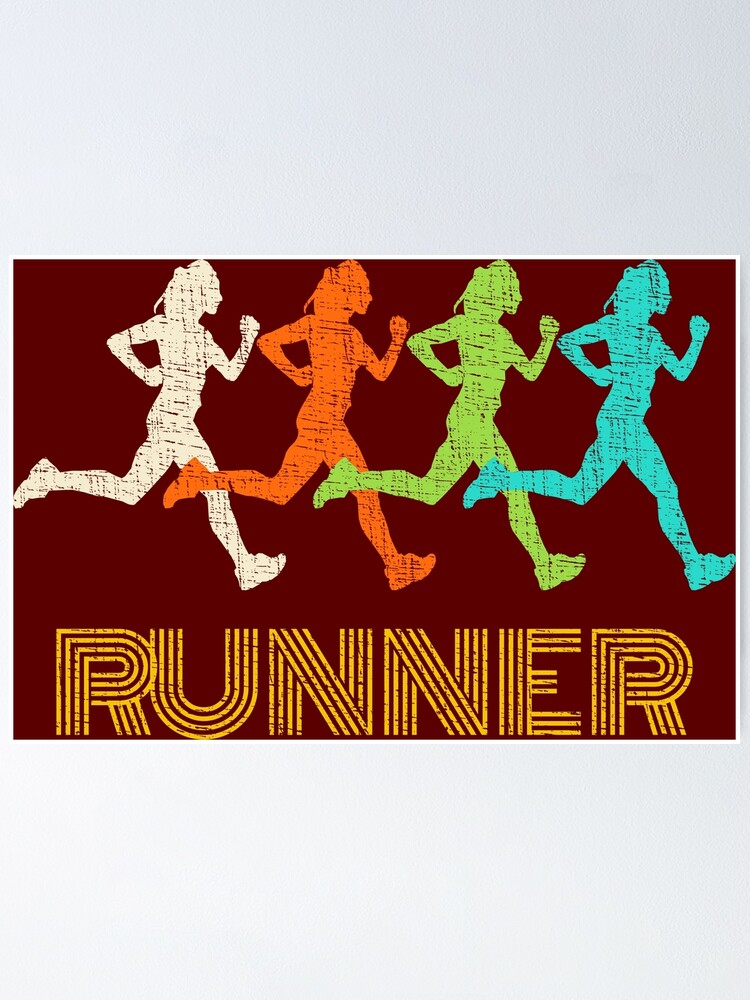The image is a postcard-shaped illustration depicting four runners, each in a different silhouette color, against a maroon-red to dark brown background. The runners, all in identical poses with left legs extended and right feet touching the ground, have their arms pumped, appearing in mid-stride. The first runner on the left is white, followed by a bright orange, then a bright green, and the last is vivid blue. At the bottom of the image, the word "RUNNER" is prominently displayed in all caps, created from yellow lines with spaces revealing the background color. Each letter is intricately composed of multiple parallel lines forming their shapes, adding a dynamic visual element to the text.